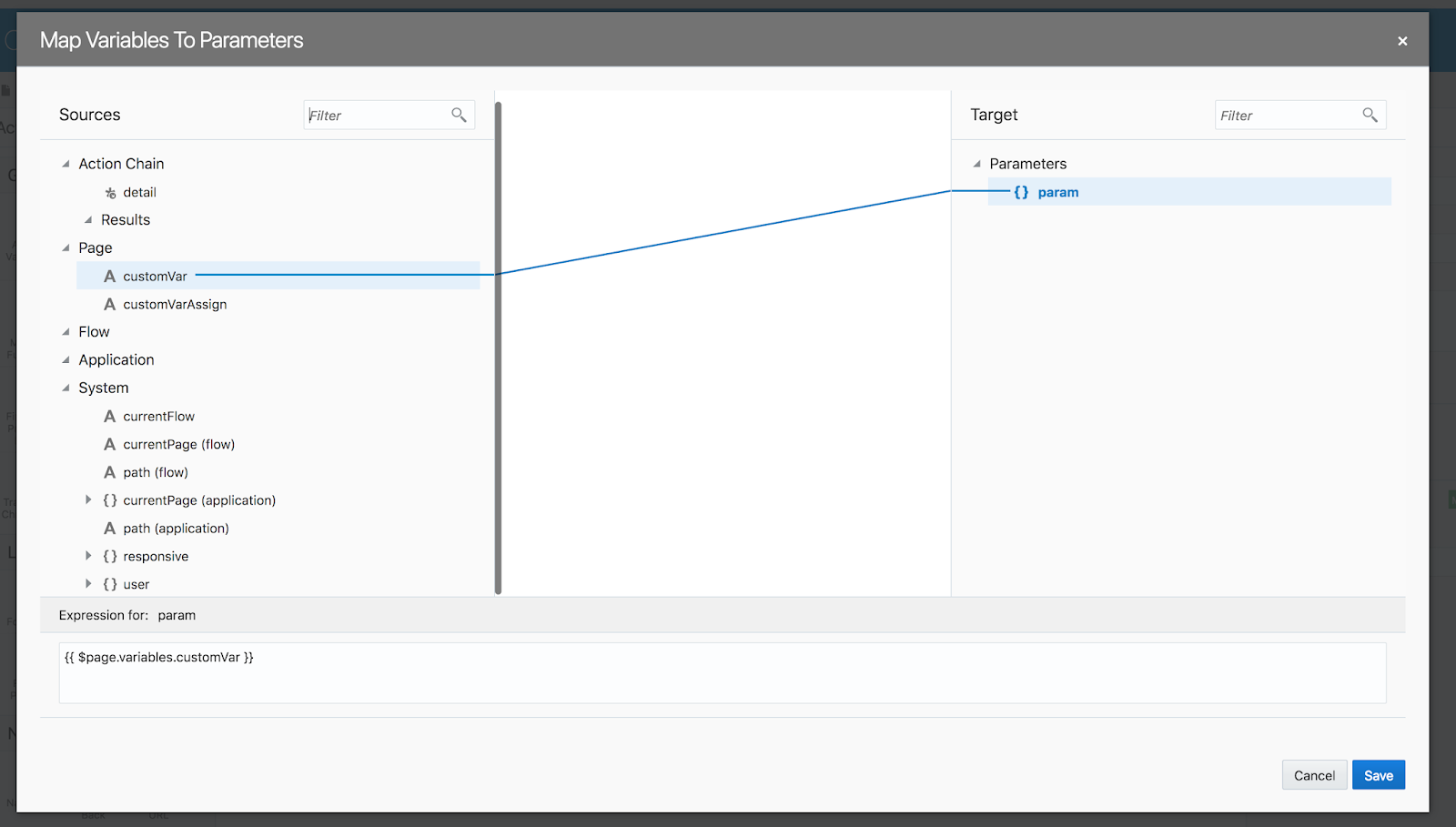This is a detailed caption for an image described via voice:

The screenshot captures a detailed interface overlay, likely from a software application focusing on data management. The top left corner features white text reading "Map Variables to Parameters," set against a gray background that extends across the top like a banner. This overlay resembles a dialog box, probably activated from the main page to allow detailed editing.

Below the banner, the interface lays out a structured grouping of categories. The initial category, labeled "Sources," lists "Action Chain." Directly beneath, it features entries: "Data," "Detail," "Results," "Page," "Customize," "Customize/Assign," "Flow," "Application," and "System." The "System" category further subdivides into three subcategories: "Current Flow," "Current Page Flow," and "Path Flow." Following this, it lists: "Current Page," "Application," "Path Application," "Response," and "User."

A subtle, curving line in the background ascends and then levels out, suggesting an underlying graphical element that might be part of the interactive elements affected by this interface overlay.